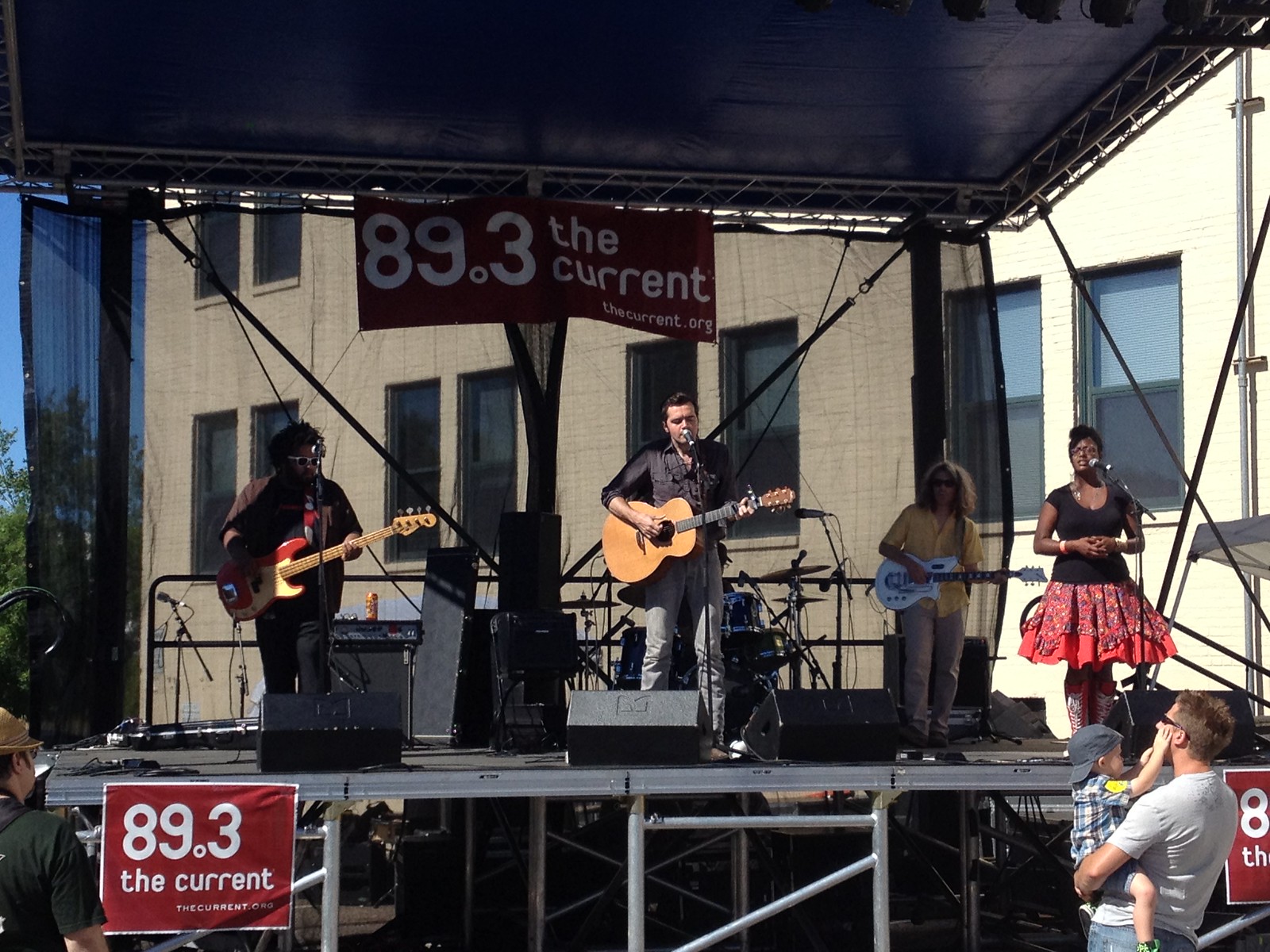This outdoor photograph captures a vibrant live performance on a constructed stage draped with banners reading "89.3 The Current" and "TheCurrent.org". The stage, situated in front of a large white building, features a canopy with a metal frame providing cover for the performers. Central to the image are four musicians: three men and one woman.

On the left side of the stage, a musician with short or medium-length curly hair, wearing sunglasses, plays an electric guitar. To the center stands the lead singer, clad in jeans, with short black hair, skillfully strumming his guitar and singing into the microphone. Slightly back and to his right, a guitarist with long blonde hair and a yellow shirt provides harmonious background tunes, adding depth to the musical ensemble. The right side of the stage showcases an African-American woman, likely the lead vocalist, wearing a short-sleeved black blouse and a striking red skirt complemented by lace-up boots. She stands poised at her microphone, hands cupped in front of her, deeply immersed in her performance.

In the audience, at ground level, two notable figures draw the eye: in the bottom right corner, a man in a gray t-shirt and blue jeans cradles a young boy who reaches endearingly for his father's face. On the left corner, another spectator, wearing a hat and shirt, watches the scene intently. The detailed setup of the stage along with the enthusiastic crowd underscores the communal and engaging atmosphere of the event.